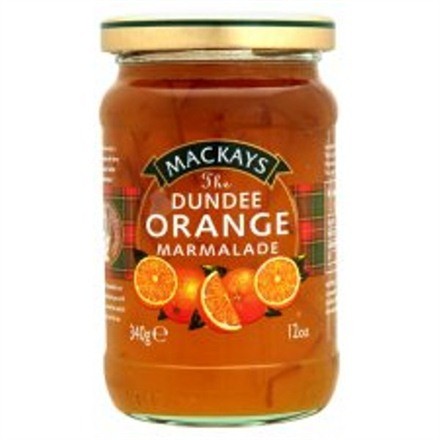This is an image of a vintage jar of McKay's Dundee Orange Marmalade. The jar itself is made of clear glass, allowing the orangish-colored marmalade inside to be visible, with a slightly darker hue at the top. The jar is topped with a gold twist-off cap. The label prominently features a black banner with "McKay's" written in bold white text. Below the banner, "Dundee Orange Marmalade" is also written in white text against the orange background of a circular design. Surrounding the text are images of oranges—two whole oranges and three slices (two halves and one segment). Flanking either side of the central label, there are tartan-patterned bands that wrap around the jar, adding a distinctive Scottish touch. The bottom of the label contains the product weight, marked as "340 grams" on the left and "12 ounces" on the right.